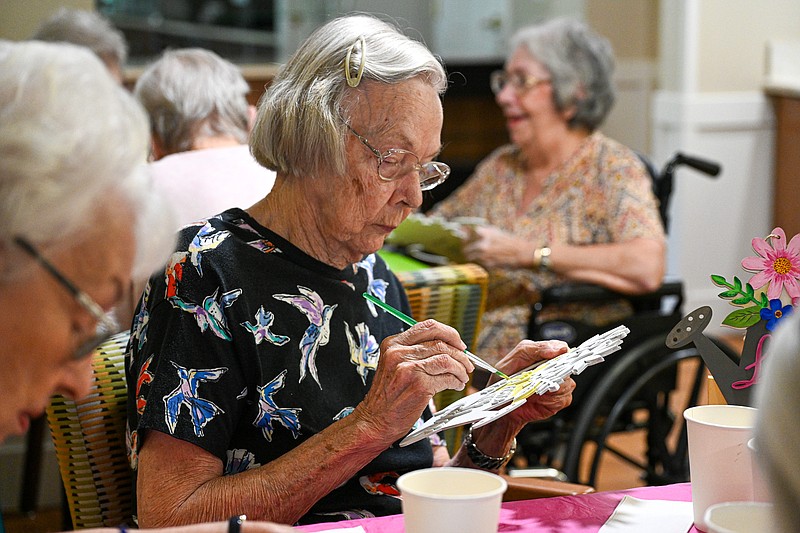The image depicts a vibrant and lively scene inside a nursing home or retirement center. The focus is on an elderly woman, who is diligently painting a cutout flower yellow with a green paintbrush. She is light-skinned, with gray hair partially tied back with a clip, and wears glasses. Her hands and face are wrinkled with age. She is dressed in a black shirt adorned with colorful hummingbirds. The table she sits at is covered with a pink tablecloth and contains paper cups possibly for rinsing brushes, along with a crafty planter's face beside her. Seated next to her is another elderly woman engrossed in her own crafting. 

In the blurred background, there is another table with at least three more elderly individuals. Among them, a cheerful woman in a wheelchair, wearing glasses, can be seen smiling and holding the same kind of craft as the woman in focus. The overall atmosphere is one of quiet concentration interspersed with moments of joy, as everyone, except the animated woman in the wheelchair who appears to be talking and laughing, is deeply engaged in their respective activities. The setting is imbued with a sense of community and creative engagement.